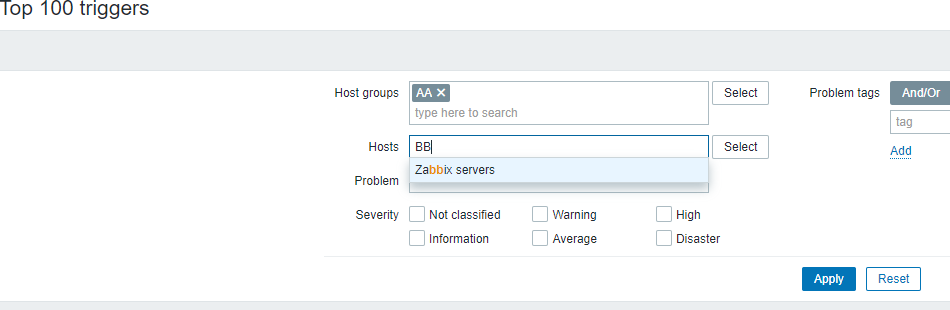The image appears to be a screenshot clipped from a desktop monitor, showcasing a section of a 1990s or early 2000s-style database interface. The primary focus is a table titled "Top 100 Triggers." The interface features a monochromatic color scheme, dominated by shades of gray, white, and light blue. 

The table contains columns labeled "Host Groups," "Hosts," "Problem," and "Severity." Under "Host Groups," there is an entry labeled "A." In the "Hosts" column, someone is in the process of typing "BB Zabbix servers." The "Severity" column has not been filled in. The interface includes "Apply" and "Reset" buttons, suggesting the user can submit or clear their inputs.

The background of the image is plain white, emphasizing the simplicity and utilitarian design of the software. The top of the interface mentions "Top 100 Triggers," although it’s unclear what this specifically refers to in the context.

Overall, the image captures a moment of interaction with a vintage database system, and judging by the context, it might be used for setting up or managing DNS or web host configurations.